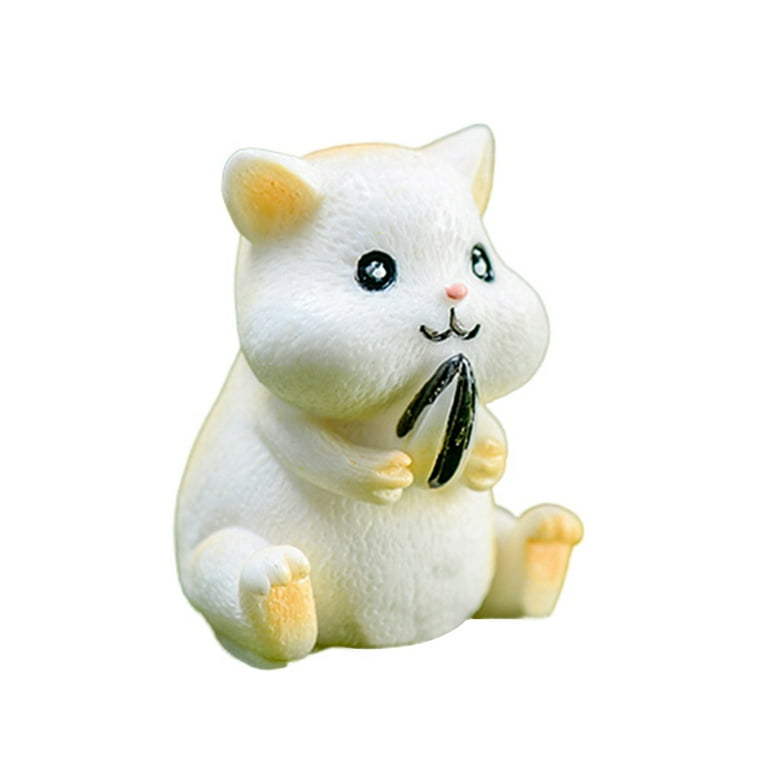The image features a figurine that appears to be either a hamster or a kitten, crafted from plastic or ceramic. The figurine is depicted in a squat, chunky form and is predominantly white with slight yellowish highlights on its feet, paws, and the inside of its ears. It has round, black eyes with tiny white dots painted inside, giving them a lifelike sparkle. The figurine also showcases puffy cheeks and a smiling expression beneath a little pink nose. It is positioned on a completely white background, further emphasizing its cute and detailed features. The creature is holding a small black object, possibly a sunflower seed or another small item, adding to its charm.